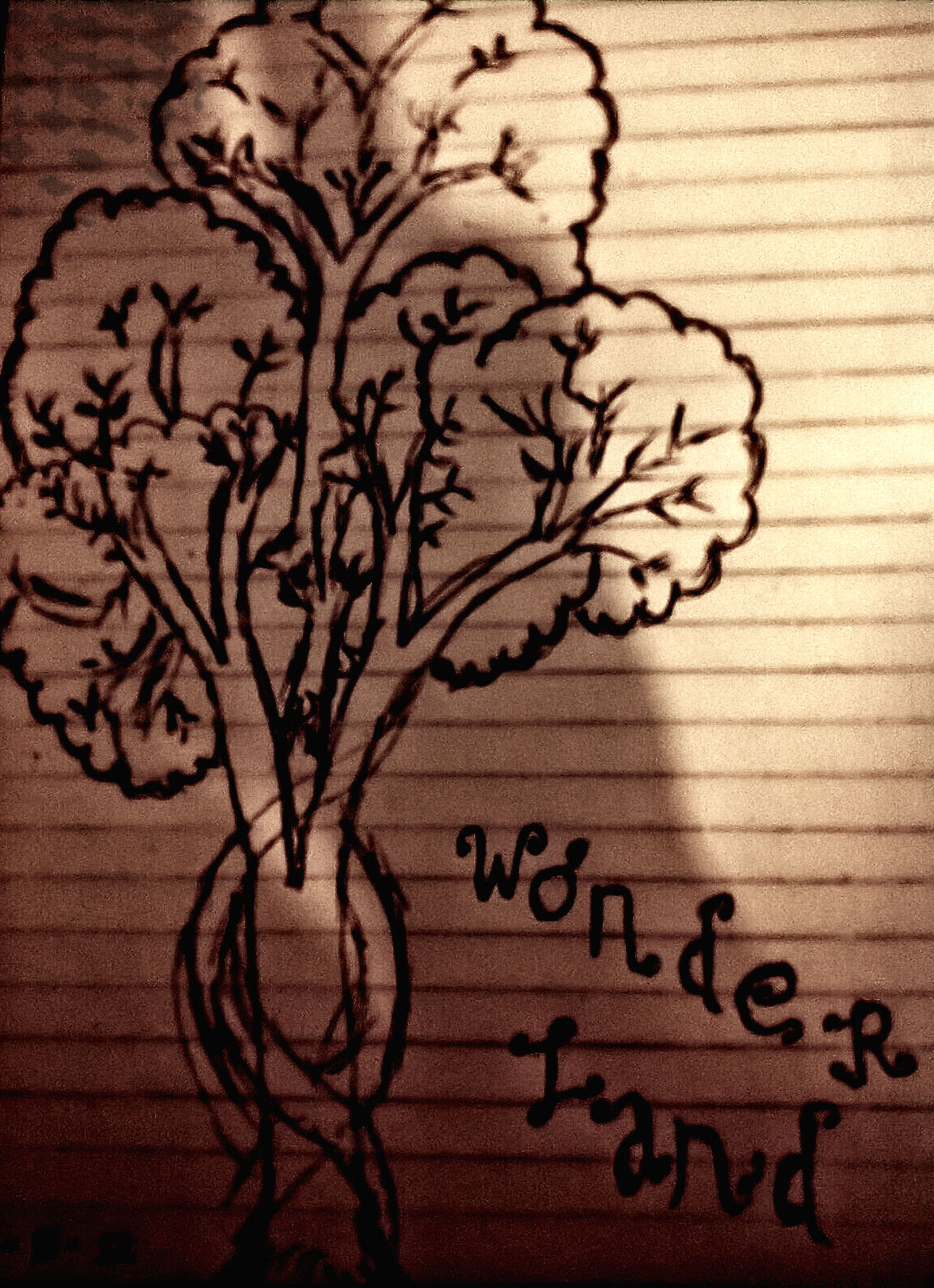The image features a white background adorned with numerous black stripes arranged in a linear pattern, giving the appearance of the paper being divided into multiple sections. In the bottom right corner, the word "Wonderland" is elegantly written in a cursive font, with the ends of the letters artistically curving outward. To the left of the text stands a tree with its tall, green leaves and bushy foliage extending upwards, creating a natural canopy. Branches from the tree spread out in various directions, intertwined with twisting vines that gracefully weave in and out of the scene, adding a whimsical touch to the overall composition.